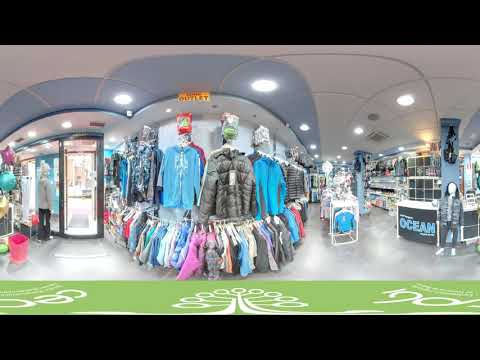This horizontally aligned, smaller-sized image depicts the interior of a clothing store with a detailed, immersive view that suggests it might be a VR or distorted perspective. The top and bottom of the image are bordered in thick black. At the very bottom, a green rug with a white pattern, possibly resembling the shape of a tree, covers part of the shiny gray tile floor. Just beyond this area, the curved rack in the center displays coats and hoodies, with more clothing items beneath it. 

A woman, possibly a customer or employee, stands on the left side, dressed in black pants and a gray top, with her long blonde hair pulled up in a bun. The scene is somewhat blurry, making her features indistinct. Near the right side of the image, a mannequin dressed in a jacket, pants, and tennis shoes stands by a column.

Text elements within the store include the word "outlet" in a yellow sign positioned at the top center and the word "ocean" near the right, adjacent to a smaller mannequin. The shop's well-lit ceiling showcases a swirled pattern of gray lines against a white backdrop. Throughout the space, winter and outdoor clothing in various colors, such as black, blue, purple, and red, are prominently displayed.